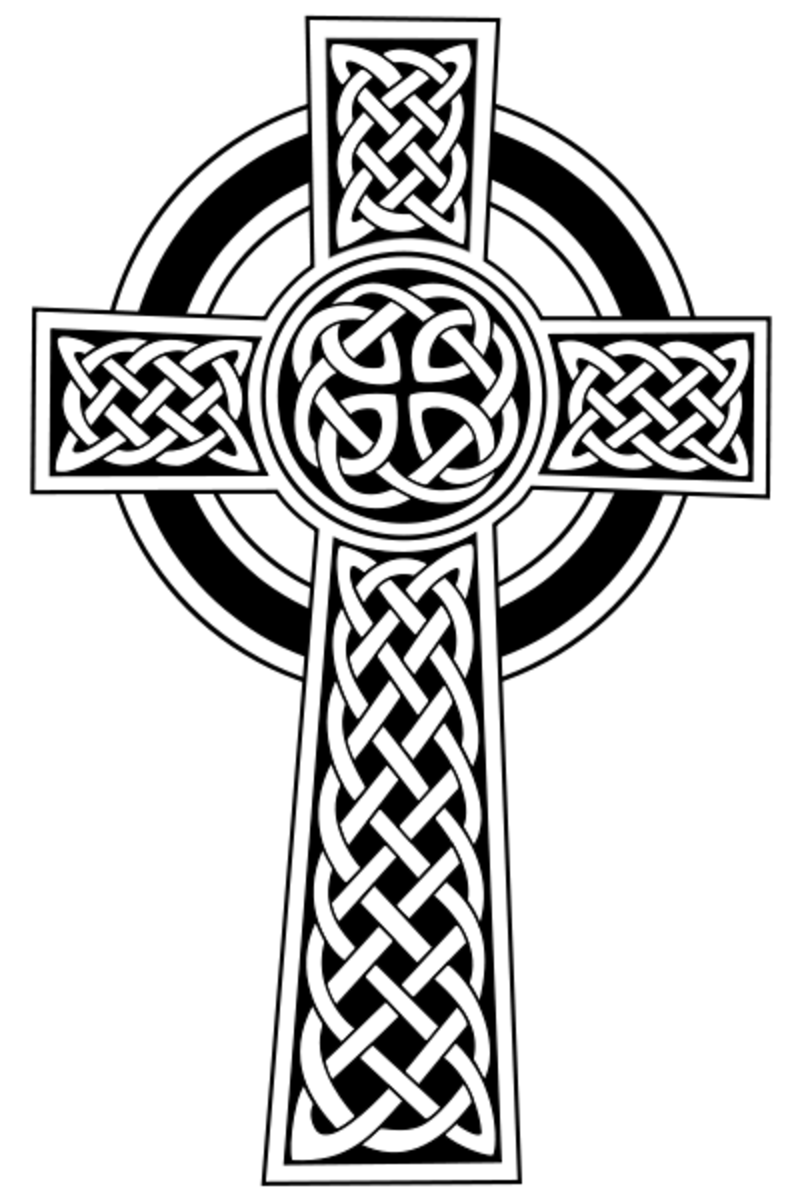The image is a detailed, black-and-white illustration featuring a central cross surrounded by intricate knot work. At the intersection points of the cross's north, east, south, and west arms, a smaller circle with interconnecting lines creates an abstract pattern. Each arm of the cross also contains this braided, woven design, giving the appearance of a tattoo. Behind the cross, there's a larger circle resembling a halo that encircles the upper half of the cross. This circle is detailed with alternating black and white inlines, adding to the intricate and artistic nature of the illustration. The background of the image is plain white, highlighting the detailed black-and-white motif of the cross and its surrounding elements.